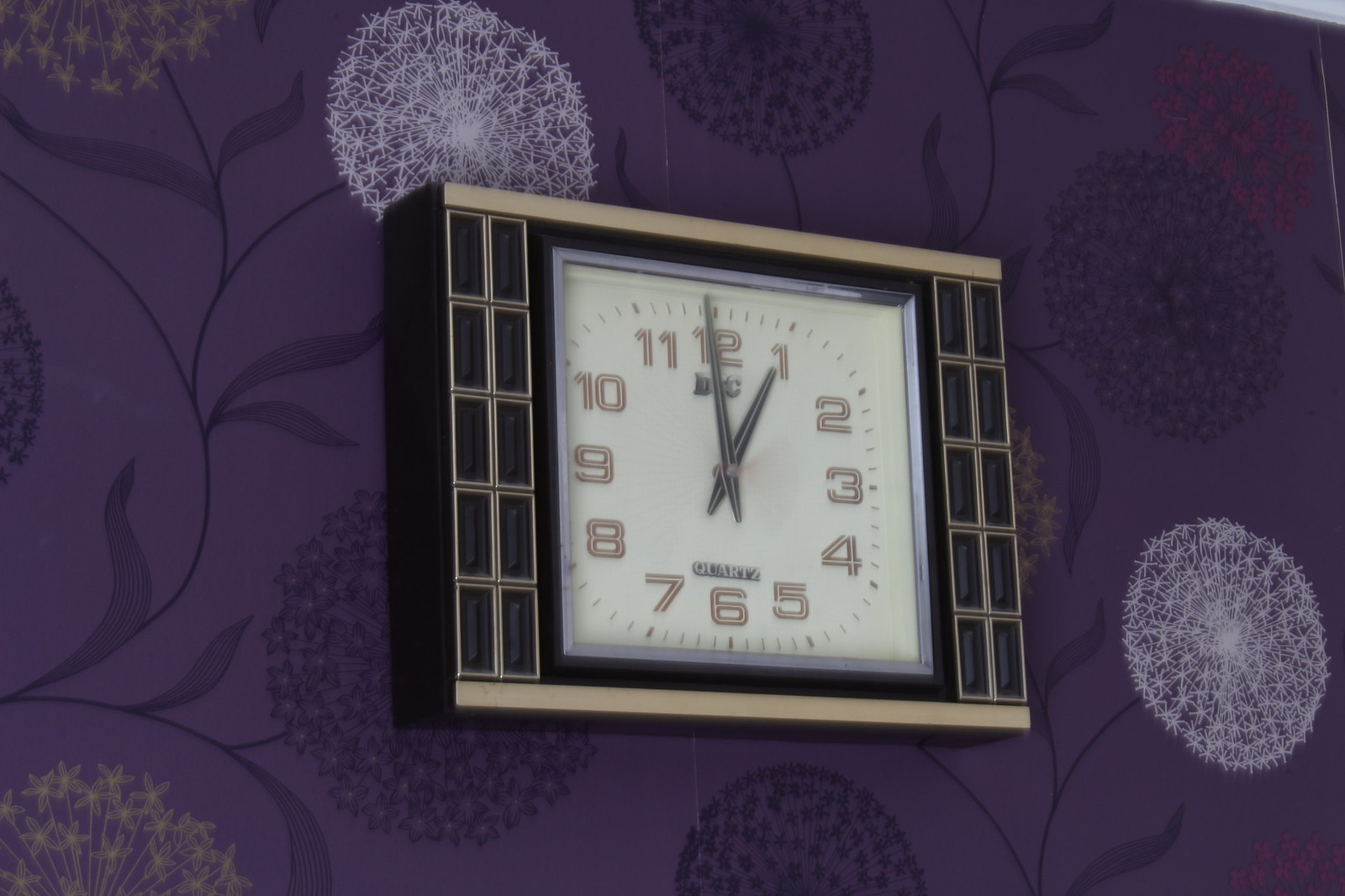The photograph features a clock mounted on a richly textured background. The background appears to be a dark purple wallpaper adorned with delicate vine-like lines and slender leaves. Embedded in the wallpaper pattern are white dandelion heads, each surrounded by fine, snow-like seeds. Notably, there are two prominent dandelion puffs: one in the upper left corner and another in the lower right corner. A hint of a yellowish dandelion head peeks out from the lower left.

Centrally placed, the clock captures attention with its elegant design. It boasts a white center adorned with gold numeral markers and black hands, all enclosed within a black body accentuated by gold highlights. Flanking either side of the clock, there are vertical stacks of clear gold-outlined rectangles, arranged five tall and two wide, adding a touch of geometric sophistication to the piece.